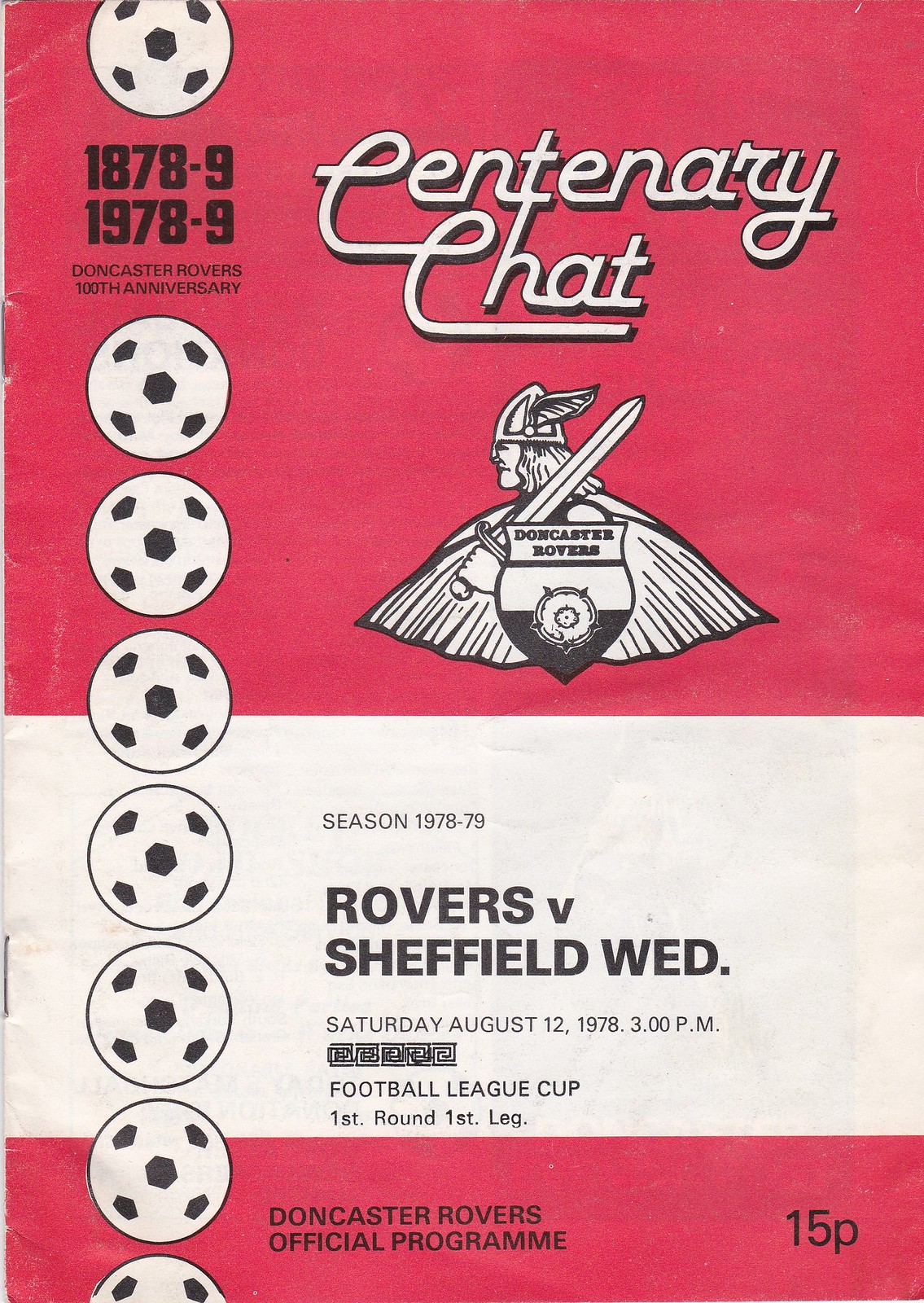This detailed image depicts a scanned cover of an official program from a historical soccer match between Doncaster Rovers and Sheffield Wednesday. The program, primarily in red, white, and black, is from the Centenary Chat marking Doncaster Rovers' 100th anniversary, dated Saturday, August 12, 1978, at 3 p.m., during the 1978-1979 Football League Cup First Round.

The cover design reflects a 1970s aesthetic, evidenced by the vintage text style, faded colors, and staple binding along the left. Down the left side, eight drawn soccer balls are present, with "1878-9, 1978-9" between the first and second, indicating the century-long history. The top section, in red, features flowing white script with a black outline reading "Centenary Chat." Below, the Doncaster Rovers' logo prominently displays a man in a Viking helmet with a sword over his shoulder set before a shield bearing a rose.

A large white stripe interrupts the red background, announcing, "Season 1978-79, Rovers v. Sheffield Wed." A complex five-part logo, somewhat unclear in detail, is positioned below, along with the context "Football League Cup, First Round, First Leg." At the bottom, a thin red stripe frames the title "Doncaster Rovers Official Program" and indicates the price: 15P.

Overall, this cover captures the essence of 1970s soccer programs, celebrating a significant milestone in Doncaster Rovers' history.